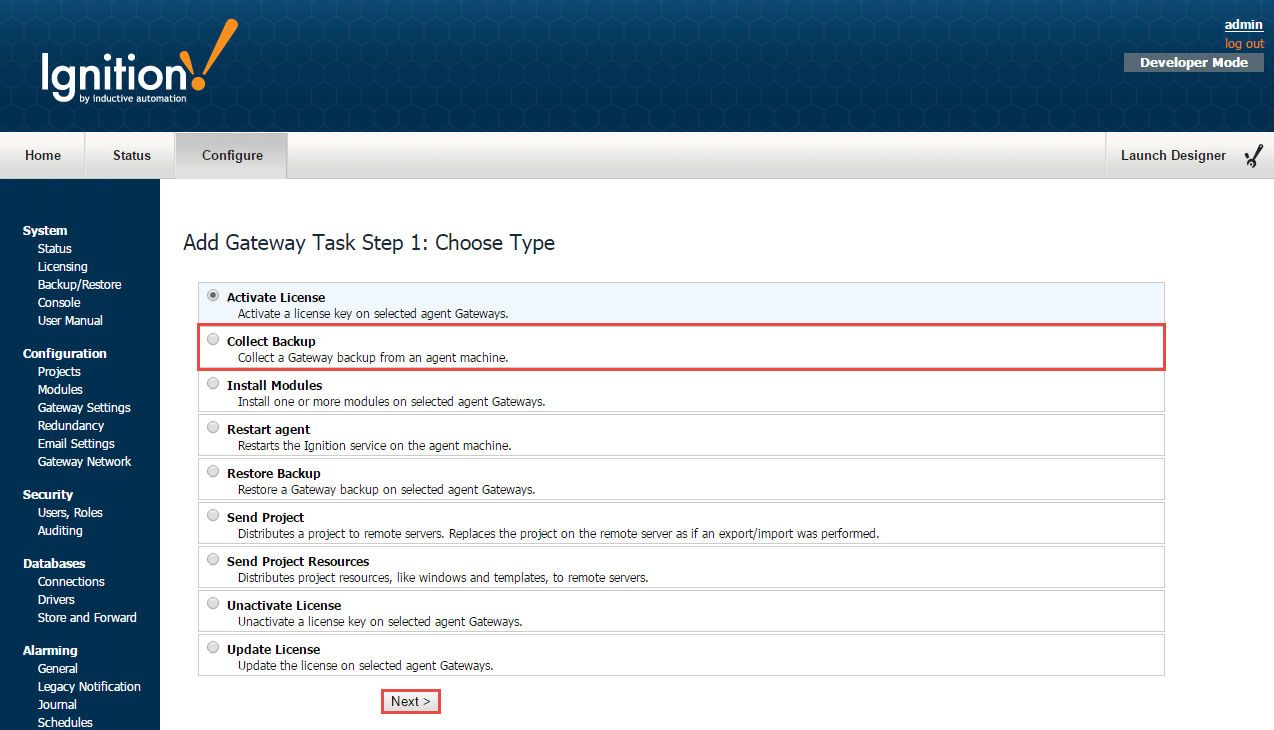The image presents a user interface for Inductive Automation's IGNITION software, against a blue background. Prominently displayed in the center is the word "IGNITION," with the subtitle "by Inductive Automation." To the right, options for "Admin Logout" and "Developer Mode" are seen, with "Logout" highlighted in orange and the other options in white.

Below, there are three primary buttons labeled "Home," "Status," and "Configure." To the right of these buttons is an option to "Launch Designer," accompanied by an icon of a wrench. To the left, situated against the blue background with white text, are several menu items including: "System Status," "Licensing," "Backup Restore," "Console," "User Manual," "Configuration," "Projects," "Modules," "Gateway Settings," "Redundancy," "Email Settings," "Gateway Network," "Security," "Users," "Roles," "Auditing," "Databases," "Connections," "Drivers," "Store and Forward," "Alarming," "General," "Legacy Notification," "Journal," and "Schedules."

To the right side of the image, there is a section titled "Add Gateway Task Step One: Choose Type," which provides a list of options:
1. Activate License: Activate a license key or selected agent gateways.
2. Collect Backup: Collect a gateway backup from an agent machine (highlighted in red).
3. Install Modules: Install one or more modules on the selected agent gateways.
4. Restart Agent: Restart the Ignition service on the agent machine.
5. Restore Backup: Restore gateway backup on selected agent gateways.
6. Send Project: Distribute a project to remote servers, replacing the project on the remote server as if an export/import was performed.
7. Send Project Resources: Distribute project resources like windows and templates to remote servers.
8. Unactivate License: Unactivate a license key on selected agent gateways.
9. Update License: Update the license on selected agent gateways.

At the bottom of this list, there is a "Next" button, which is also highlighted in red.